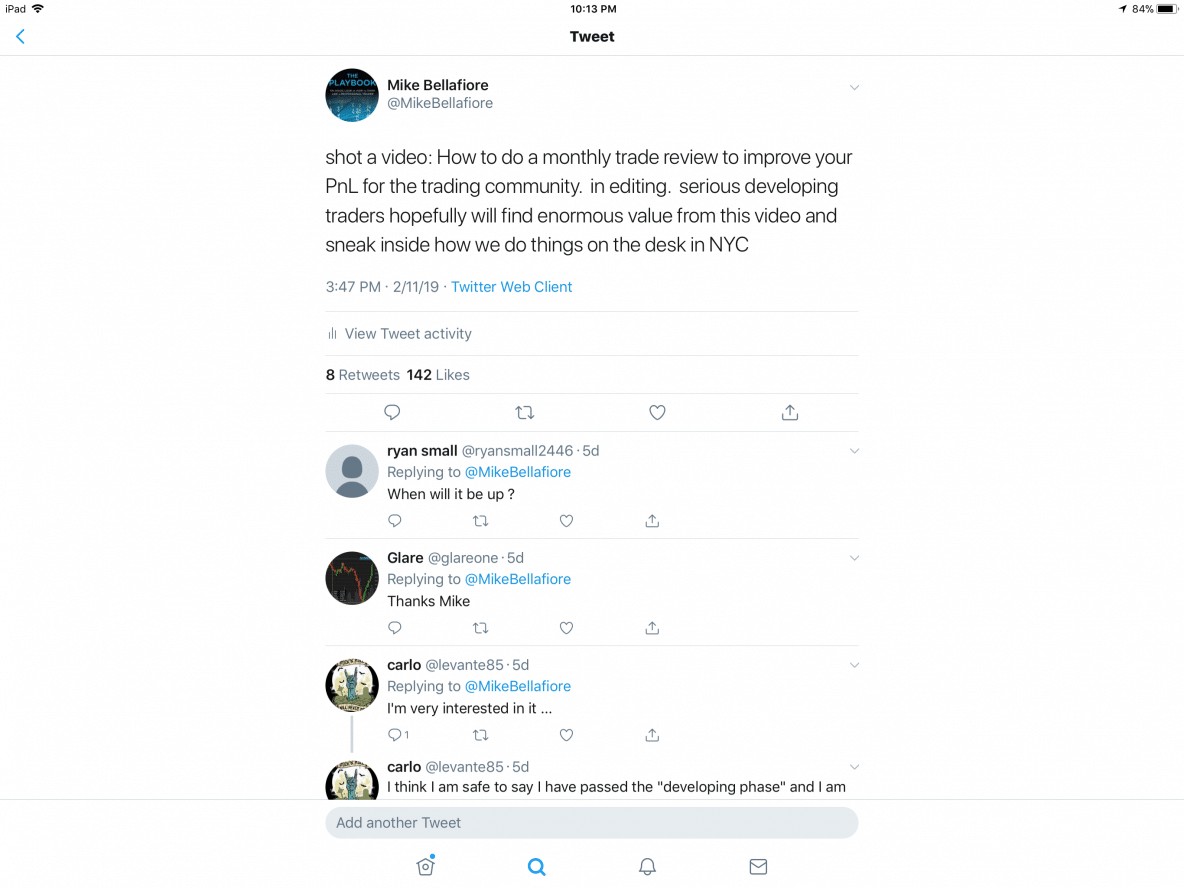**Detailed Caption:**

A screenshot captured on an iPad at 10:13 PM depicts a tweet from Mike Bellafiore posted at 3:47 PM on February 11th, 2019, using the Twitter web client. In the tweet, Mike mentions that he shot a video explaining how to conduct a monthly trade review aimed at improving P&L (Profit and Loss) for the trading community. He emphasizes that serious and developing traders will hopefully find immense value in the video and get an insider's look at the trading processes on his desk in NYC. The tweet received significant engagement, including 8 retweets and 142 likes.

Several replies to the tweet express keen interest:
- Ryan Small asks, "When will it be up?"
- A user named Glare thanks Mike.
- Carlo comments twice, expressing his interest and confidence that he has moved past the developing phase, although his second comment cuts off abruptly.

The screenshot also shows Twitter's interface at the bottom, including the homepage, search, notifications, and inbox icons. This level of engagement highlights why users post on platforms like Twitter—to garner interest, involvement, and interaction from their audience regarding their activities and content. Mike's initiative to share educational content and behind-the-scenes insights is well-received and contributes to fostering a connected community.